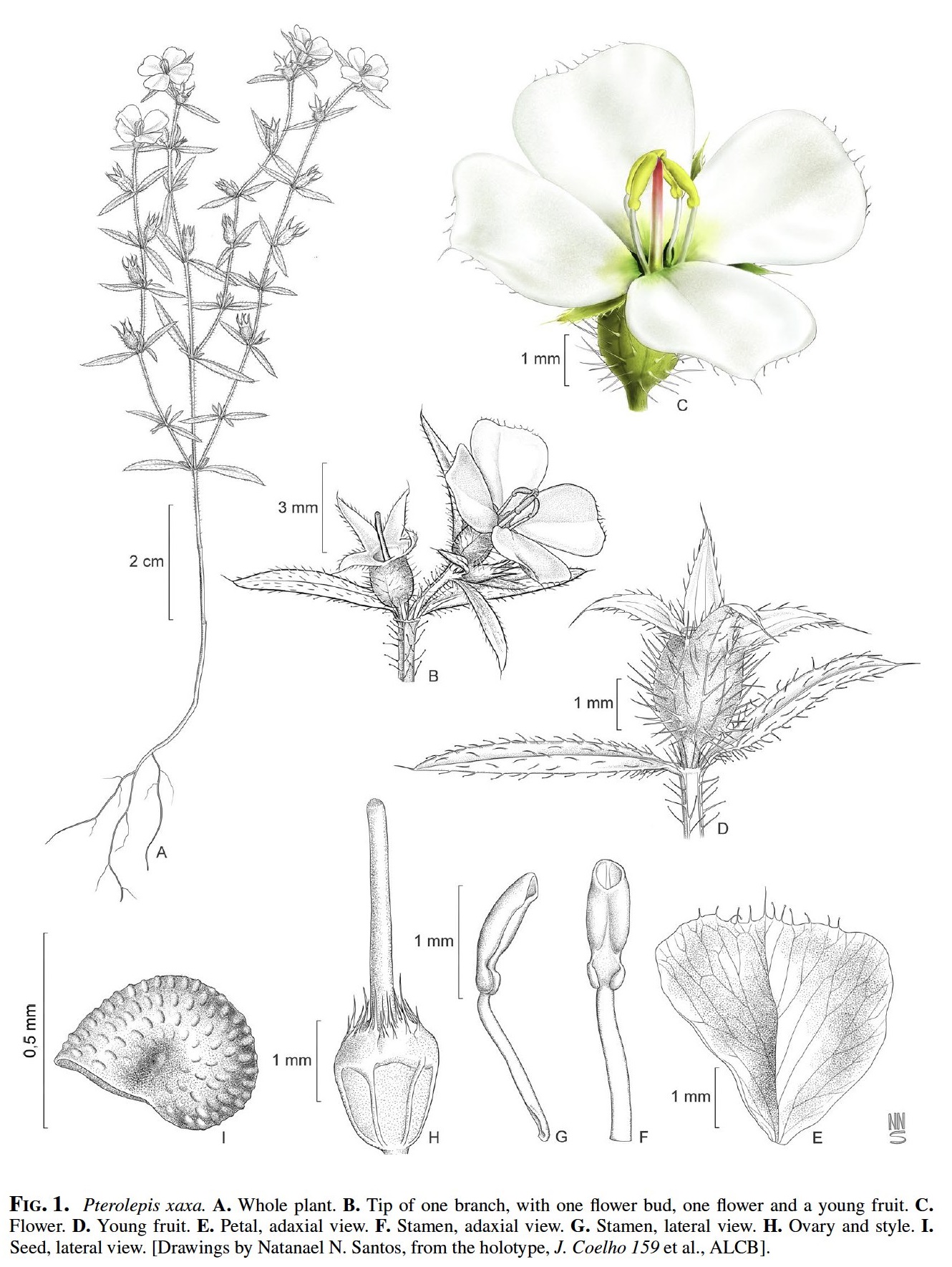This image appears to be a detailed scientific diagram from a book, illustrating various parts and stages of a flower's development. Dominating the upper section is a colored depiction of a flower in full bloom, featuring four white petals with spiked tips, a yellow center speckled with a hint of pink, and a green stem. This is the only colored segment in an otherwise monochromatic array of sketches.

Surrounding this central bloom are multiple black and white illustrations, each meticulously labeled from A to I. These sketches include a range of botanical elements: a leafy plant with small flowers, the tip of a branch with a flower bud, an open flower alongside a young fruit, isolated petals, the stamen in both frontal and lateral views, the ovary and style, and a seed from a lateral perspective. Each drawing is scaled with measurements, commonly noted as one millimeter. 

At the bottom of the diagram, a legend provides scientific terminologies for the various parts depicted above, offering a reference for understanding the intricate details of each labeled section.